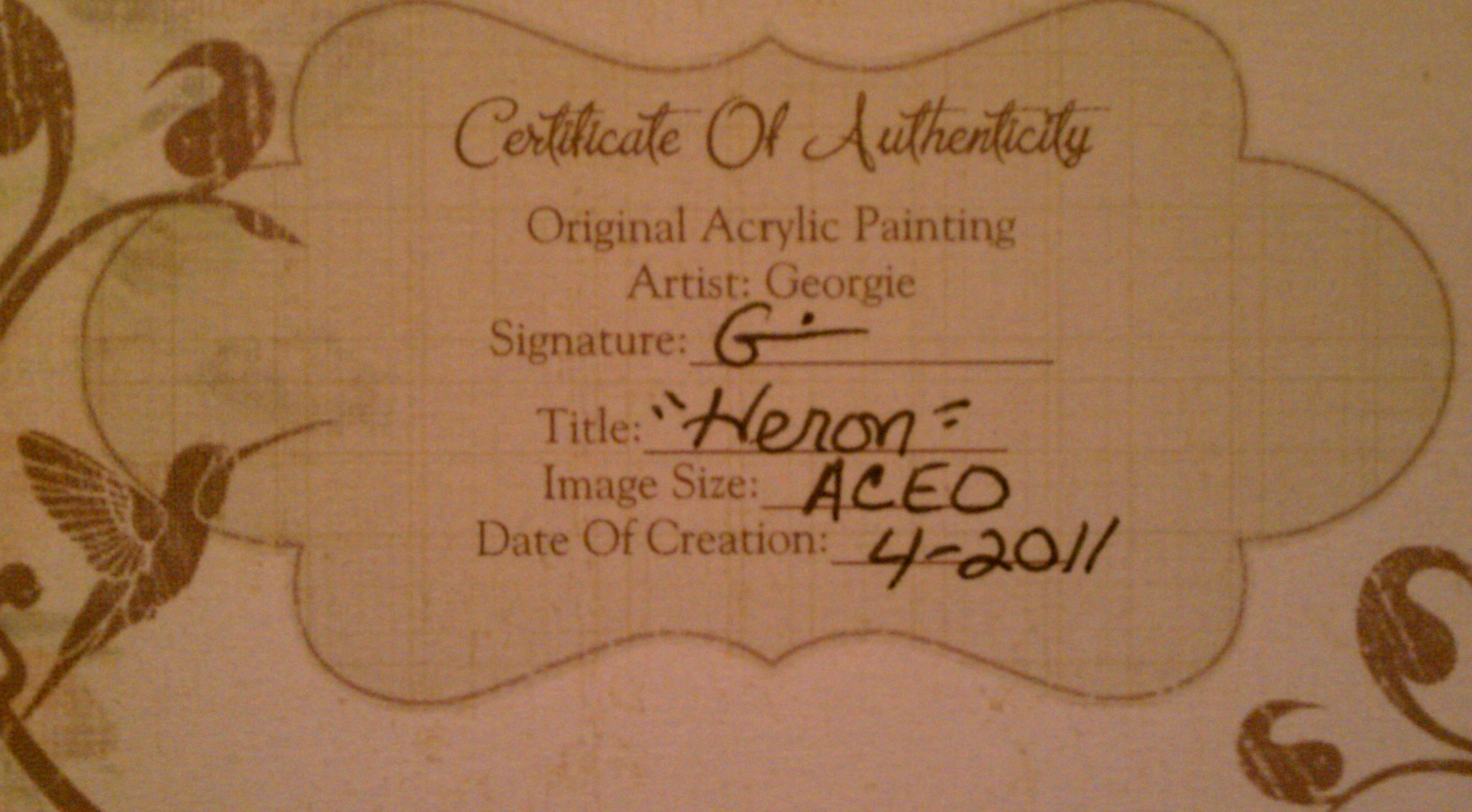This photograph depicts a detailed Certificate of Authenticity presented on a thick, light brown piece of paper. The text at the top reads "Certificate of Authenticity" in cursive red letters, followed by "Original Acrylic Painting" in a similar style but with a Times New Roman-like font. The text continues with "Artist Georgie," and "Signature," which features a handwritten 'G' in black ink. The title section notes the artwork as "Heron" (H-E-R-O-N) also in quotes and black ink. The "Image Size" is indicated as "A-C-E-O" and the "Date of Creation" reads "4-4-2011."

The design of the certificate includes various graphic details such as a red silhouette of a hummingbird in the bottom left corner, floral decorations on the left and lower right sides, and additional floral elements depicted as stems and leaves in the upper left and lower right corners in brown. The overall aesthetic combines both printed and handwritten elements to create an authentic and visually appealing document.